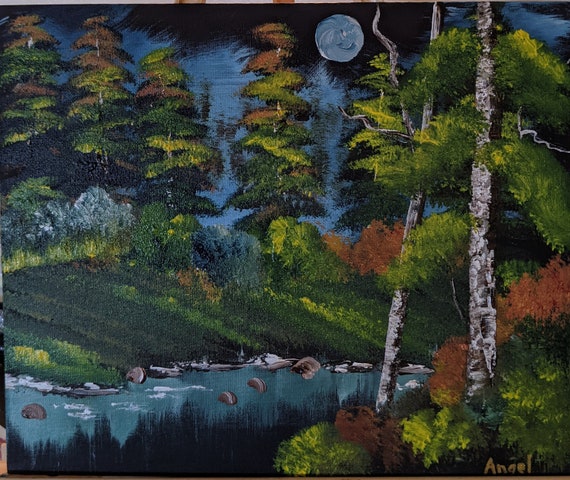This painting depicts a serene nighttime forest scene centered around a gently flowing river or creek. The river, reflecting the night sky's gradients of dark blues and blacks, has light ripples with white caps and contains gray rocks. Tall evergreen trees, likely pine, with rich green foliage and some scattered brown leaves, flank both sides of the river. The striking whitish-gray trunks of birch trees add texture and interest, with their green leaves contrasting the scene. Near the riverbank, a mixture of light and dark green grass, along with orange and green brushes, suggests a lush undergrowth. The ground also features various small bushes in shades of orange and green. Above the landscape, the sky transitions from dark black to lighter blue hues, punctuated by a light blue moon almost in the upper middle right. The painting’s broad strokes and smudgy appearance suggest it might be an oil painting, and despite not being the work of a master, it carries a charming, rustic quality. At the bottom right corner, the artist's name, Angel, is signed in brown, completing this tranquil riverscape.